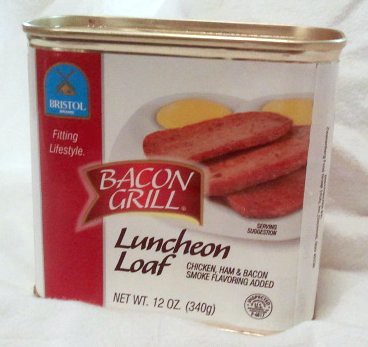A can of potted meat, designed in a rounded rectangular shape with smooth, curved corners. The top of the can features a metallic gold tin lid. Encircling the sides is a label that prominently displays a sleek color scheme of black, red, and white. The front of the can is adorned with a detailed image of neatly sliced portions of the potted meat, providing a visual representation of the product inside.